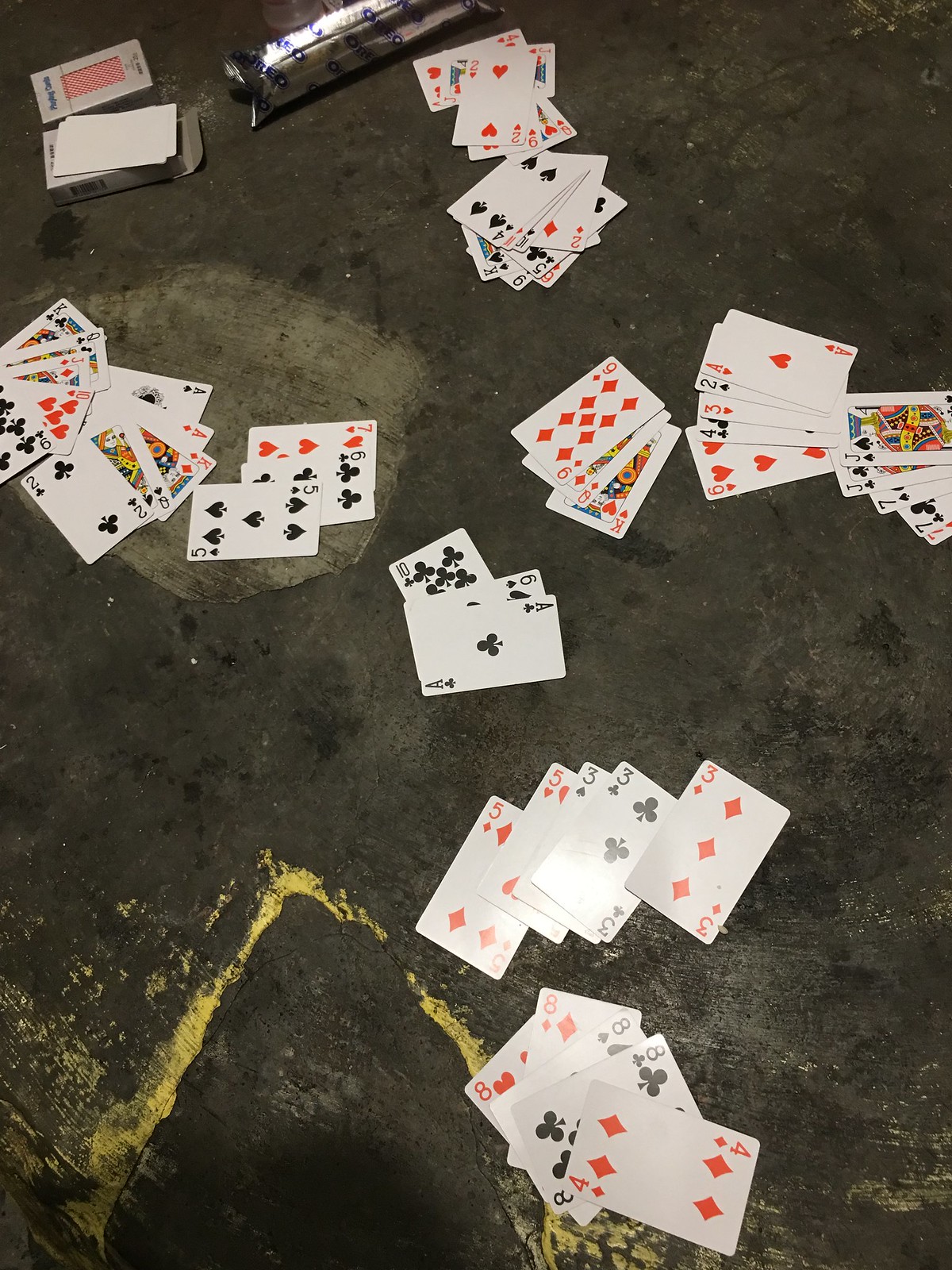A chaotic scene of white playing cards scattered haphazardly across a dirty concrete ground adorned with visible yellow cracks. The cards are strewn in various piles with some discernible groupings: 

- At the bottom is a pile consisting of the four eighths and above them, the four of diamonds.
- Another pile contains the two fives, five of diamonds, five of hearts, three of spades, three of clubs, and three of diamonds.
- Centrally located in the image, there is a pile featuring the ten of clubs, six of spades, and ace of clubs.
- Right above this, a group includes the nine of diamonds, queen of diamonds, and king of hearts.
- To the right, a pile holds the six of hearts, four of clubs, three of hearts, two of spades, and ace of hearts.
- Further right, the collection shows the seven of hearts, seven of clubs, seven of spades, another seven of clubs, jack of clubs, and jack of spades.
- Towards the top of the image, numerous cards are present but indistinct.
- More towards the upper left is the seven of hearts, six of clubs, and five of spades.
- To the left of this grouping is another random assortment of cards that are hard to distinguish.

This scattered and disorganized assembly of cards creates a visually striking contrast against the gritty, cracked concrete background.